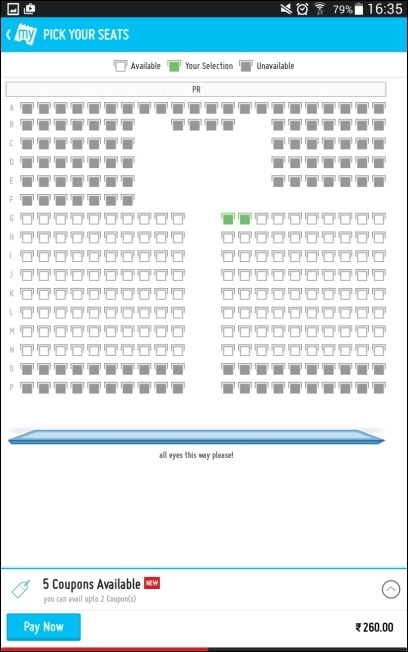The image is a screenshot from a mobile phone. In the top right corner, it displays the time as 16:35, with the phone battery at 79% charge. The status icons show the Wi-Fi signal, an alarm clock, and the phone is on mute. The main part of the image features a website for a concert venue’s seating selection.

At the top of the website, there is a prompt that reads "Pick Your Seats" with a left-pointing arrow indicating a back function. Below it are several icons: a legend for available seats, a green icon indicating your current selection, and a dark gray square showing unavailable seats.

The seating chart of the venue is displayed, showing rows labeled from A to P. Rows A to F and rows O and P are all grayed out, indicating these seats are unavailable. The remaining rows in the middle are available for selection. Two seats in row G, located in the second half of the section, are currently selected. The total cost for these two seats is $260. At the bottom left of the screen, there's a prominent blue button labeled "Pay Now" for purchasing the selected seats.